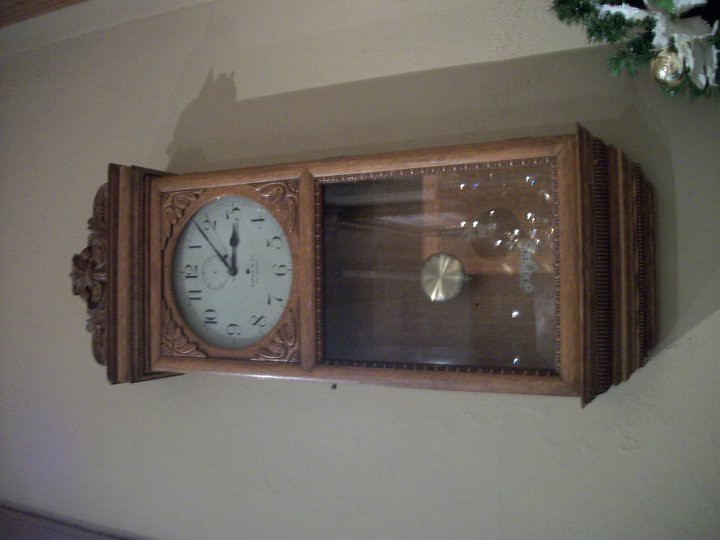The photograph depicts a grandfather clock hanging on a beige or white drywall, with the image captured horizontally, necessitating a 90-degree turn for proper viewing. The clock features a light brown wooden frame with intricate engravings, lending it an elegant appearance. At the top of the clock is a fancy logo, followed by a circular clock face with an off-white background and black numerals arranged clockwise. The long black hand points between 1 and 2, while the short hand points to 3, indicating the time as approximately 3:08. Below the clock face is a large glass section through which a gold pendulum is visible. Near the bottom right of the image, there is a table or surface featuring what appears to be a small bouquet and some decorative items, including a bell and Christmas decoration.